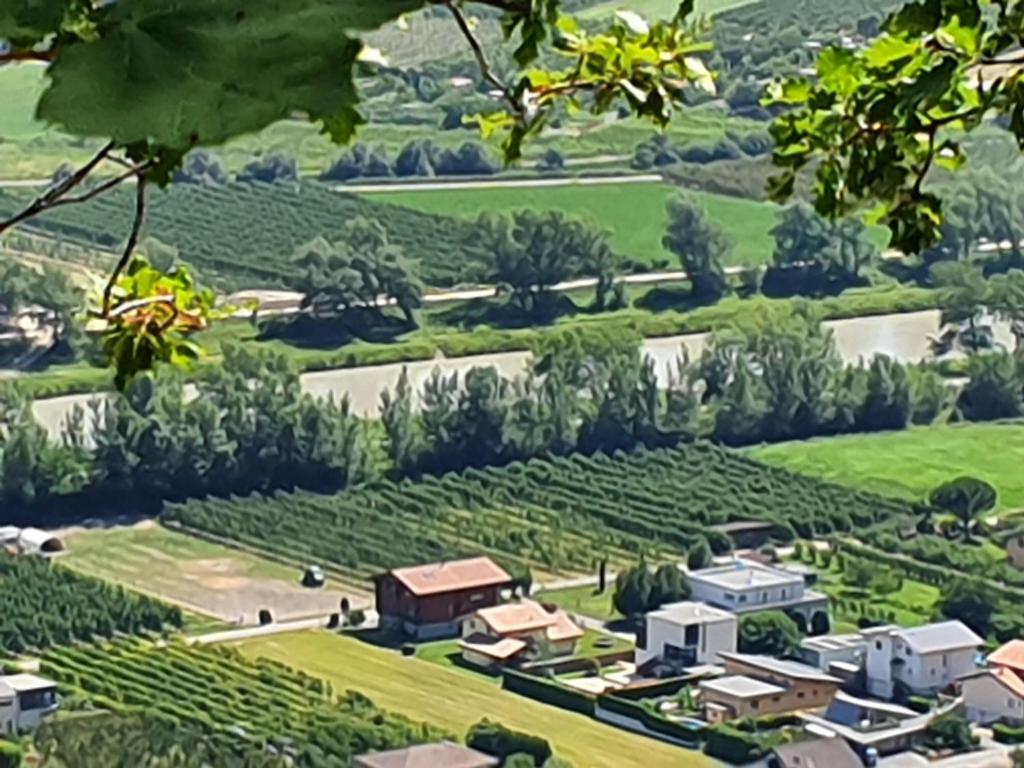This aerial photograph showcases a picturesque blend of farmland and a small rural neighborhood. In the foreground, numerous rectangular buildings, primarily houses with a mix of pointed orange and flat white roofs, are neatly aligned, suggesting a modest town or community. Flanked by a green yard, these houses cluster along a winding road that weaves its way through the predominantly grassy plain.

The landscape is meticulously segmented into different sections, each designated for various crop plantations. Verdant fields stretch across the terrain, characterized by orderly rows of crops and irrigation lines. A significant feature of the image is a horizontal body of water, possibly a canal or creek, bordered by lush trees that runs through the center.

In the background, rolling hills adorned with dense forests rise up, painting a serene picture of nature's bounty. The farthest section of the image reveals the foothills of majestic mountains, their green slopes dotted with occasional structures. The scene is imbued with extensive greenery, showcasing different shades of cultivated vegetation, and capturing the tranquil beauty of agricultural life.